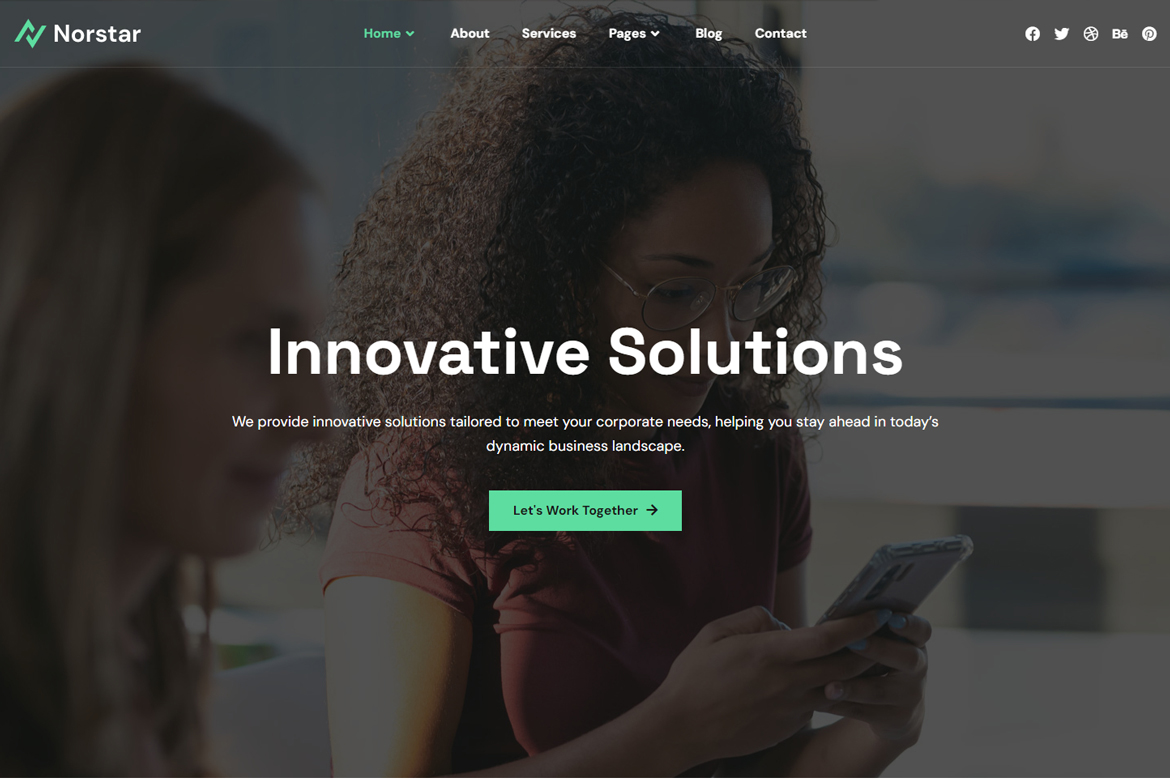An image from OR Star Innovative Solutions features two women in the background, each engrossed in their respective phones. The scene captures a bustling environment where technology and communication are at the forefront, illustrating the company's commitment to modern and innovative approaches in business. The subtle details of the setting suggest a dynamic and forward-thinking atmosphere, emblematic of OR Star's dedication to cutting-edge solutions.